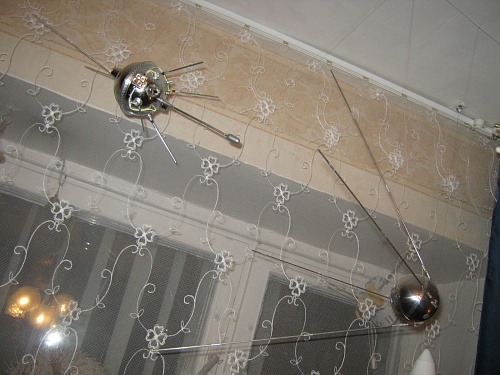The image depicts a unique and slightly dated living room setting with a focus on two decorative art pieces resembling space probes. The main subjects are two round golden spheres, each adorned with multiple antenna-like legs, suspended from the ceiling by nearly invisible wires, likely made of fish wire. The orb on the right has four long antenna legs, while the one on the left sports at least seven. These intricate sculptures are evocative of old-fashioned satellites. In the background, the wall meets a white ceiling, decorated with a white track that supports net curtains featuring a delicate lace design with a floral pattern. Through the net, white window frames of what seem to be either windows or possibly sliding glass doors are visible, providing a glimpse of blinds behind them. The overall composition is accentuated by the white and neutral tones of the ceiling and the curtain, giving the room an airy yet nostalgic atmosphere.